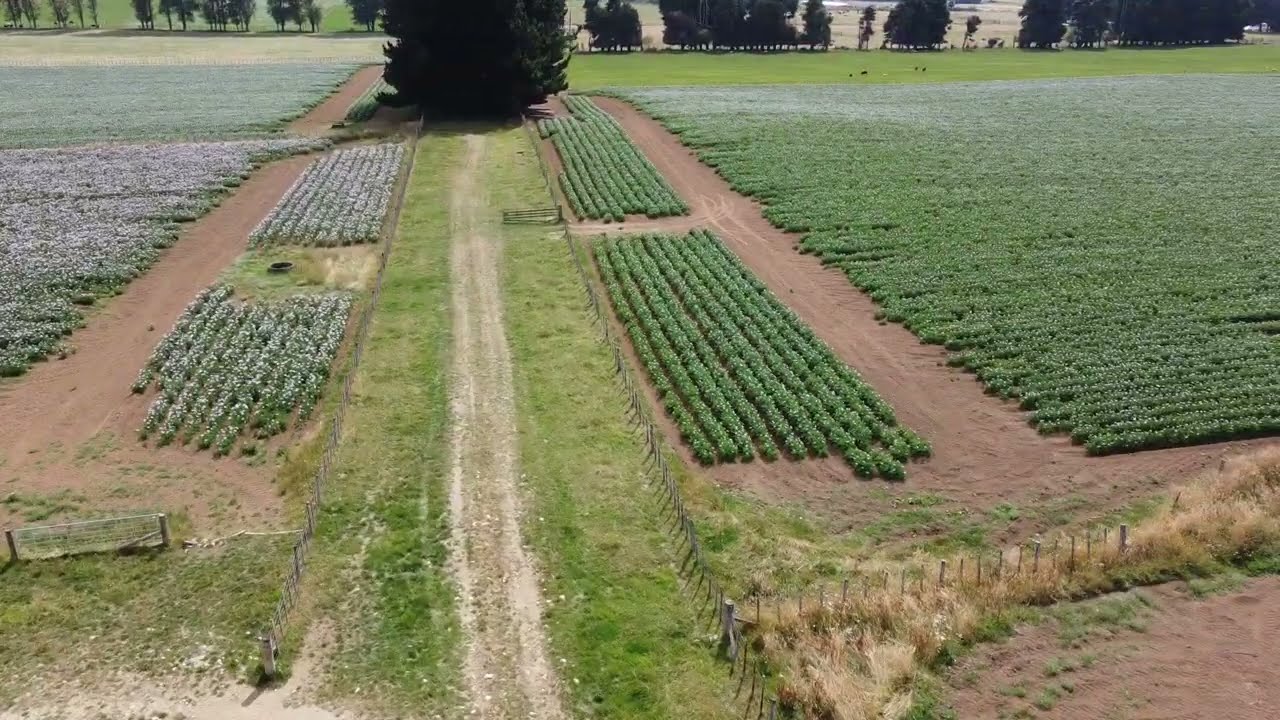The aerial photograph depicts a vibrant and expansive farming area, showcasing a lush and meticulously arranged landscape. Dominating the center is a light gray grass-patch path that stretches vertically from the bottom to the top of the image, ending at a large, bushy green tree. The path is flanked on both sides by sections of green fields, which give way to various cultivated plant rows. On the right side of the central path, a wooden fence borders the area, beyond which linear patches of vegetation are visible, some adorned with delicate purple flowers. Similarly, to the left of the path, more rows of plants, also displaying hints of purple blossoms, extend horizontally and vertically. A brown dirt path runs parallel to these sections. The horizon in the background is decorated with a scattered line of trees. The overall scene, captured in landscape orientation, is a harmonious blend of various shades of green and showcases the structured beauty of agricultural land.